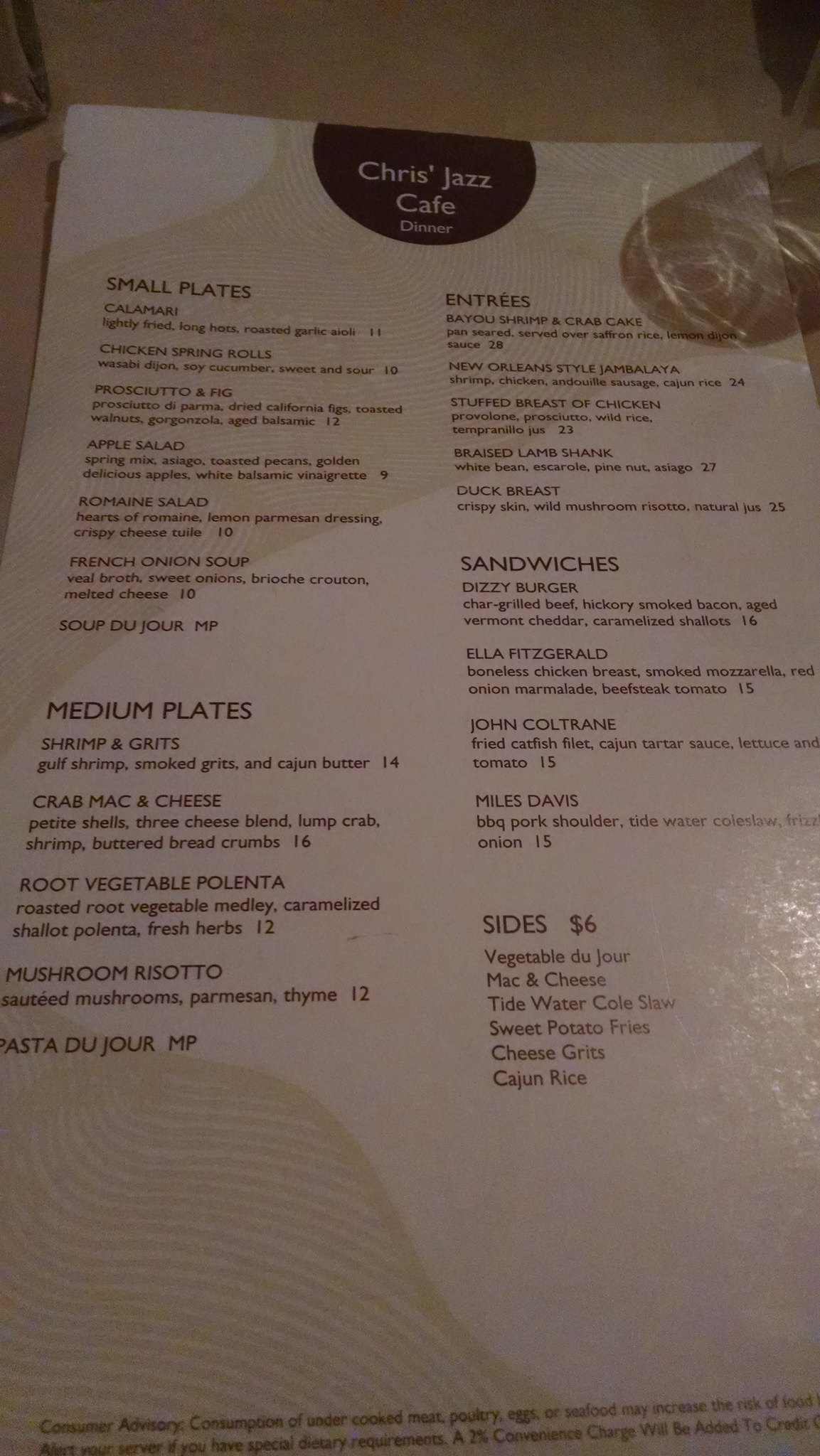This color photograph captures a dimly lit section of a menu, which appears in a muted gray tone due to the low lighting. The backdrop, slightly darker gray, peeks through at the very top of the image. In the upper right-hand corner, a water glass sits partially on the menu, casting a shadow that stretches towards the left.

The menu showcases fine print, rendering the text difficult to decipher. At the top is a black semi-circular logo next to the restaurant's name, "Chris's Jazz Cafe." The menu is organized into two columns. The left column starts with the section "Small Plates," followed by "Medium Plates." The right column features "Sandwiches" at the top, with a section titled "Sides" below, where the price "$6" is partially visible, although the specifics of the sides remain unreadable.